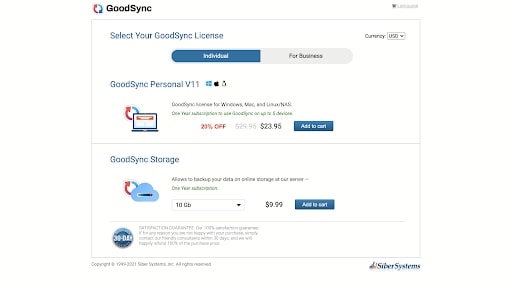The image depicts an online store interface for purchasing Goodsink storage services. At the top of the image, the title "Goodsink" is prominently displayed. Below this title, there are two distinct rectangular sections, each detailing different purchasing options related to Goodsink.

The first rectangular box is labeled "Select Your Goodsink License" and offers two options: individual or business. It features the product "Goodsink Personal V11" accompanied by logos for Microsoft and Apple, indicating compatibility with both platforms. An icon representing a computer with a circular arrow in blue and red suggests synchronization or backup features. The product is currently on sale, with a 20% discount advertised, reducing the price to $23.95. There is a clear "Add to Cart" button provided for this purchase.

The second rectangular box is dedicated to "Goodsink Storage," which includes an icon of a cloud with a circular arrow behind it, symbolizing cloud storage and data synchronization. The default storage option is 10 gigabytes, but a drop-down menu indicates the availability of additional storage options. The price for the default 10 gigabytes of storage is listed at $9.99. This section also includes an "Add to Cart" button, making it easy for users to purchase additional storage space.

Overall, the interface is user-friendly, with clear sections for different product offerings and convenient options to add selected services to the cart for purchase.